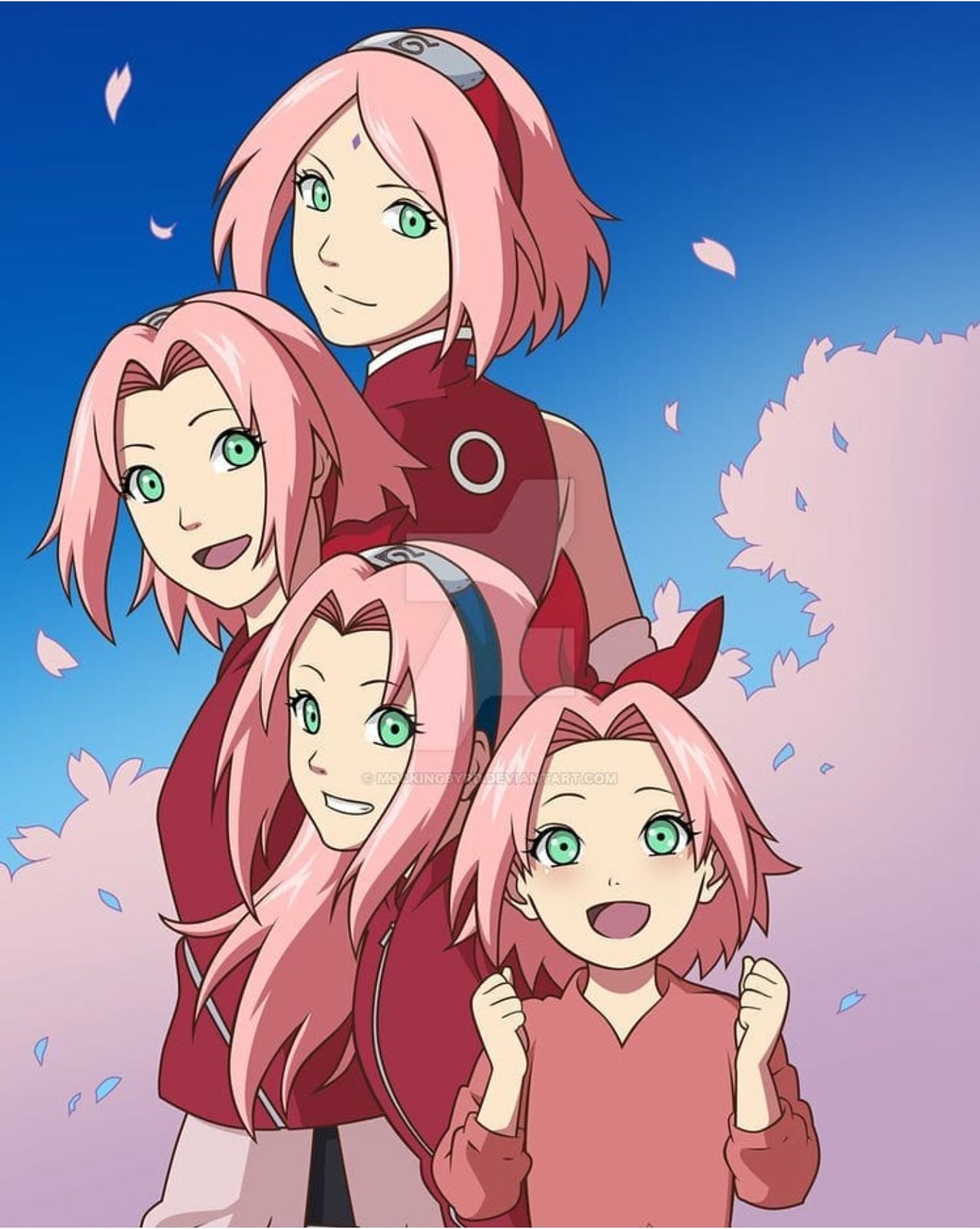The image portrays a Japanese-style manga scene featuring a family of four girls lined up by age. The eldest girl stands at the back, followed by the next oldest, a preteen, and a very young toddler positioned at the front. Uniquely, all four girls sport pink hair and striking green eyes. They wear coordinated uniforms in shades of purple and pink, with the three older girls donning headbands, while the youngest sports a bow tie in her hair. The setting is vibrant, with a clear blue sky and bushes behind them. Leaves drift through the air, suggesting a gentle breeze. The eldest girl's uniform features a plain circle logo on the back, adding a subtle detail to the scene.